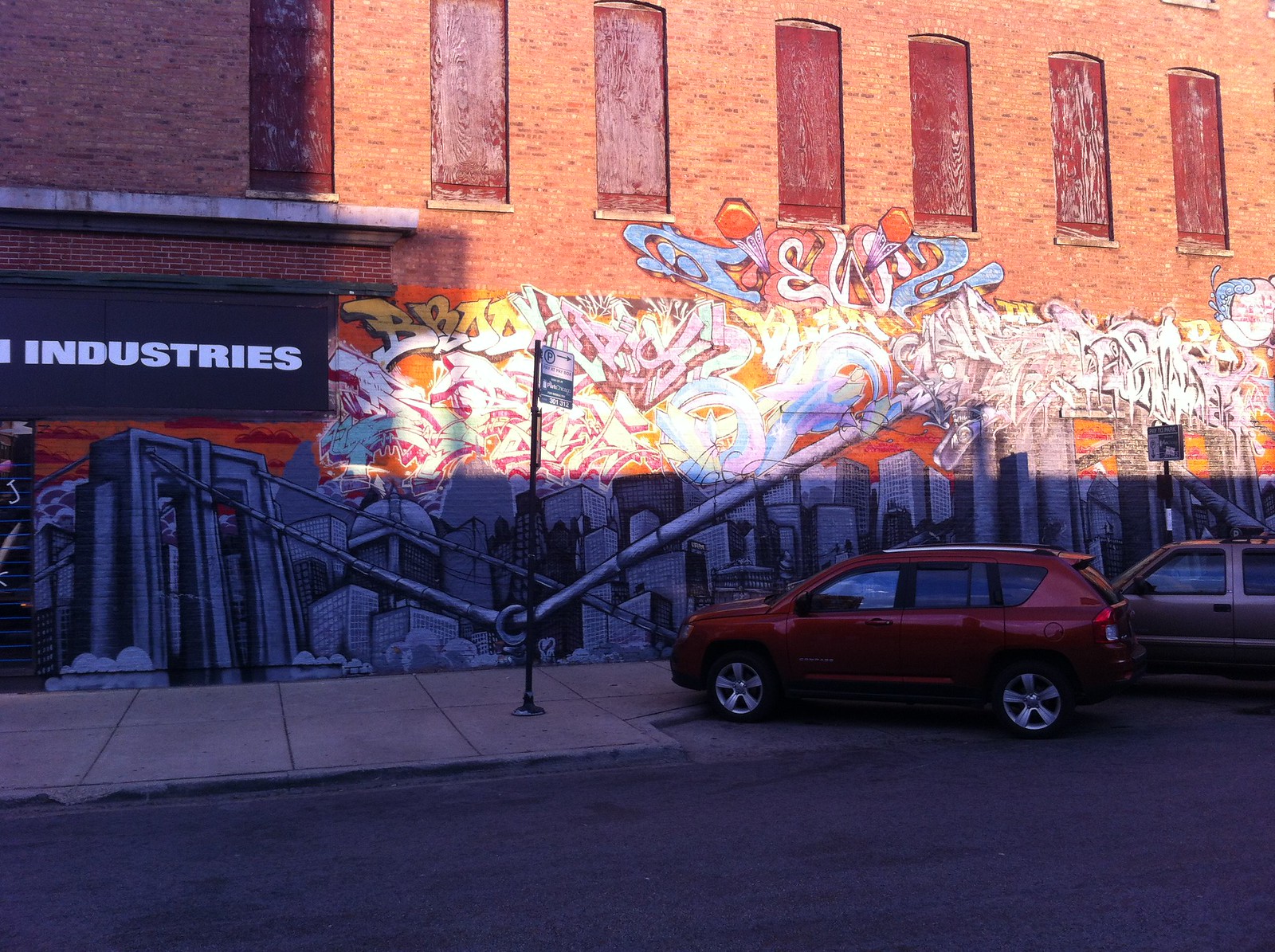The image depicts a red small SUV parked on an asphalt street in front of a red brick building, with a brown small SUV partially visible next to it. The building appears old and possibly abandoned, characterized by windows boarded up with reddish wooden planks. A concrete sidewalk separates the building from the street. The building's façade features extensive graffiti art, including multicolored tagging and a mural that depicts a cityscape with skyscrapers. On the left side of the building, a sign in white text reads "Industries," though part of the text is cut off. Additional street signs, including one black with unidentifiable text and another white and blue, are present near the parked vehicles. The road curves slightly where the vehicles are positioned.